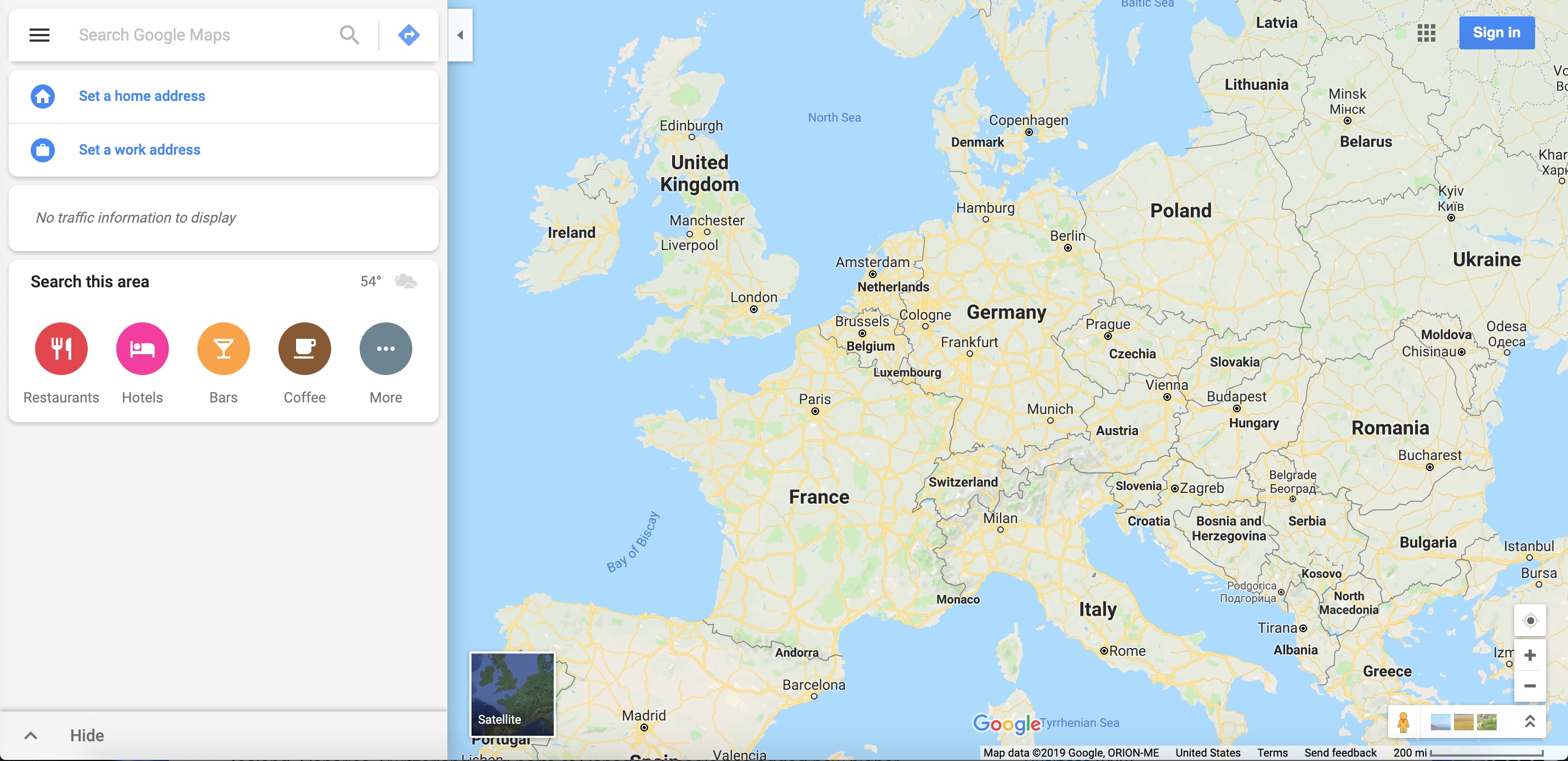In this image, a map serves as the backdrop, with various geographical locations prominently displayed. To the left, a sidebar lists several text options including "Search Google Maps," "Set a home address," and "Set a work address." It also mentions, "No traffic information to display," and provides search categories such as "Search this area," "Restaurants," "Hotels," "Bars," "Coffee," and "Mall."

Popular locations highlighted on the map include Edinburgh, United Kingdom; Manchester; Liverpool; Ireland; North Sea; Denmark; Copenhagen; Hamburg; Poland; Berlin, Germany; France; Slovakia; Romania; Bucharest; Bulgaria; Italy; Rome; Monaco; Albania; Tirana; Greece; Serbia; Hungary; Vienna; Zagreb; and Prague.

At the bottom of the image, there is a note stating "Map data © 2019 Google" and the name "Ryan Dashme."